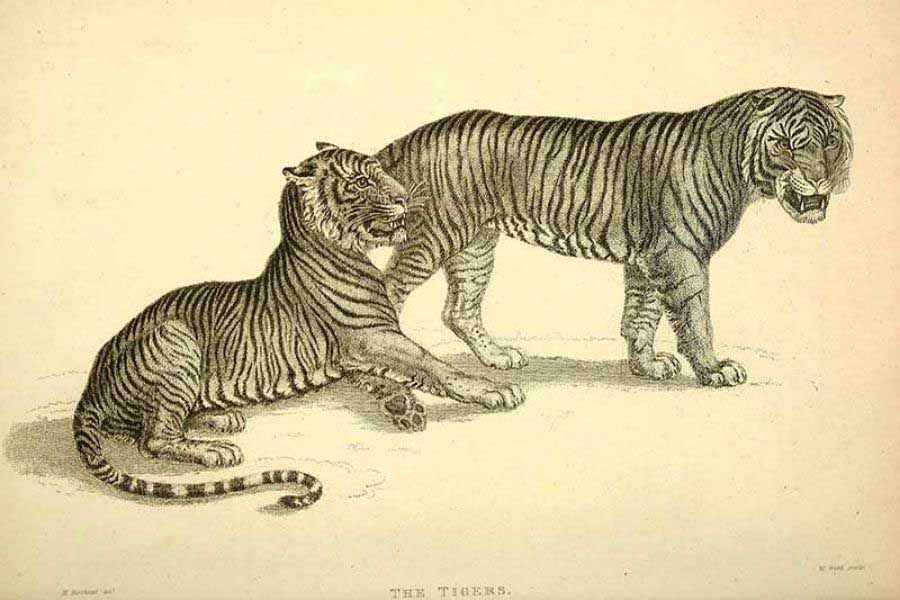This is a black-and-white illustration, possibly an etching or pen and ink drawing, of two tigers on a cream-colored, slightly yellowed background. The image is titled "The Tigers." The first tiger is prominently displayed, standing on all fours with dense black stripes and a snarl on its face, facing to the right of the image. This tiger's head is on the far right, and its body extends toward the center of the image. The second tiger lies in front of the first, stretching its front legs and appearing more relaxed. Positioned to the left, this tiger's head is near the standing tiger's hindquarters, partially obscuring its tail. The lying tiger, with a long, thin tail featuring circular stripes, also has its mouth open, displaying its teeth. Both tigers have small ears and distinctive coats with intricate line details. The overall style of the artwork resembles that of Albrecht Dürer, and at the bottom of the image, the title "The Tigers" is inscribed in light pencil.